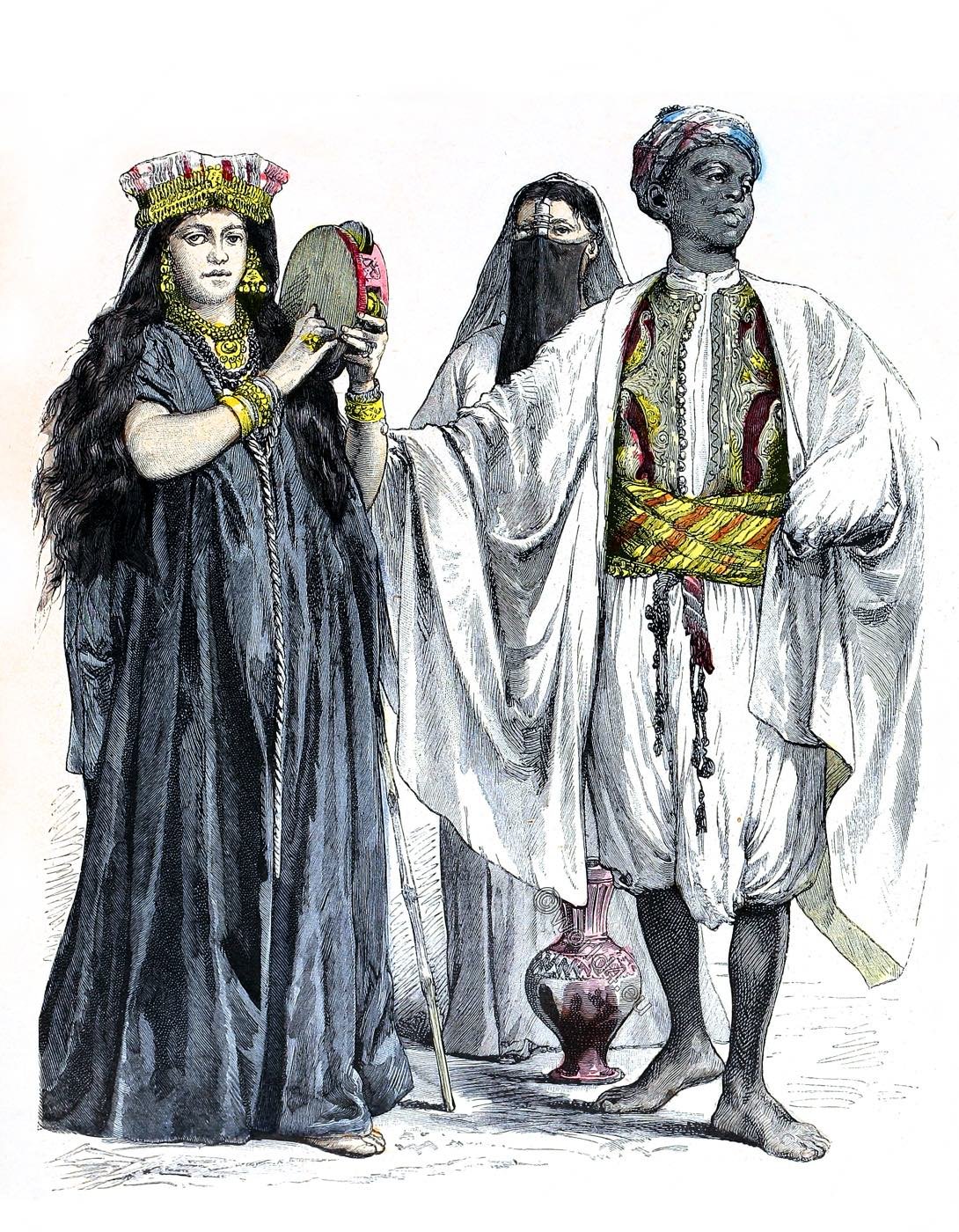This detailed hand-drawn lithograph, meticulously hand-painted, portrays three Middle Eastern individuals in traditional attire, reminiscent of a time at least 200 years ago. At the forefront, a woman stands out in a long, navy blue, short-sleeved dress that covers her entirely except for one sandal-clad foot peeking out. She boasts flowing, waist-length black hair, adorned with a gold and white hat, and is heavily accessorized with large gold earrings, an ornate gold necklace, numerous bracelets, and rings. She holds a red tambourine with a white center, posed as if in mid-performance.

Beside her, a man dressed in a white jumpsuit that stops at his knees is visible, completed with a voluminous shawl draped over his shoulders. His attire is accentuated by a colorful vest in shades of red, yellow, and white, and a striped cummerbund tied around his waist. He wears a blue, red, and white turban and stands barefoot, his darker skin contrasting with the others. He gently holds the tambourine woman's arm, looking thoughtfully to the right.

In the background, a woman garbed in a long white gown is partially obscured. Her hair is pulled back, concealed under a simple white cloth that rests on her head. Her face is mostly hidden by a black mask, revealing only her eyes and a bit of her forehead, adding an air of mystery. Adjacent details include a pink, intricately designed vase on the ground and a discreet cane leaning against the woman with the tambourine, suggesting subtle interactions among the trio. This illustration, evocative of an 1800s history book, captures an intricate moment frozen in time.